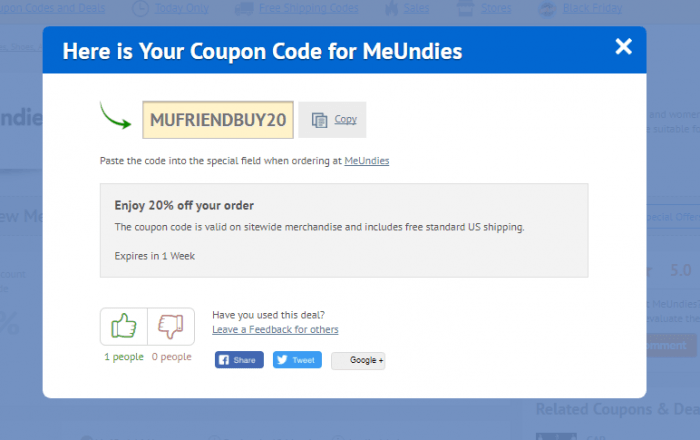The image depicts a pop-up window designed to deliver a coupon code. The window features a blue header bar with white text, aligned to the left, that reads: "Here is your coupon code for MeUndies." Just below this text, a green arrow, situated on the left side, points towards a tan-colored block. This block contains the coupon code "MUFRIENDBUY20" displayed in all capital letters with a gray font. Positioned to the right of the code is a "Copy" button, allowing users to easily copy the code to their clipboard. Further down, instructional text advises users to "Paste the code into the special field when ordering at MeUndies." At the bottom of the pop-up, a gray box announces "Enjoy 20% off your order," providing an additional incentive for customers to use the provided code.